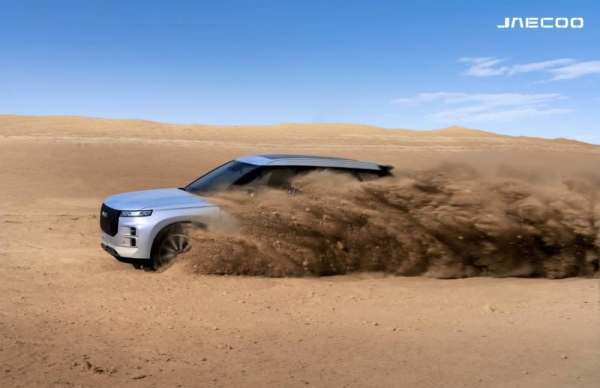The photograph captures a dynamic and thrilling scene of a silver mid-sized SUV racing through a vast, sandy desert landscape. The SUV is centered in the frame, with sand billowing dramatically behind it, illustrating its high speed and the rugged terrain. The background is a seamless expanse of desert sand that blends into a blue sky adorned with white clouds. The desert is devoid of vegetation or other obstructions, emphasizing the isolated yet adventurous setting. The SUV's tires, roof, and front hood are clearly visible, along with a sunroof, hinting at its sophisticated design. A notable feature is the text "J-N-E-C-O-O" in the top right corner, possibly the brand or an advertisement headline, lending a commercial aura to the image. This simple yet powerful scene focuses solely on the SUV conquering the sandy dunes, highlighting its capability and durability in harsh environments.